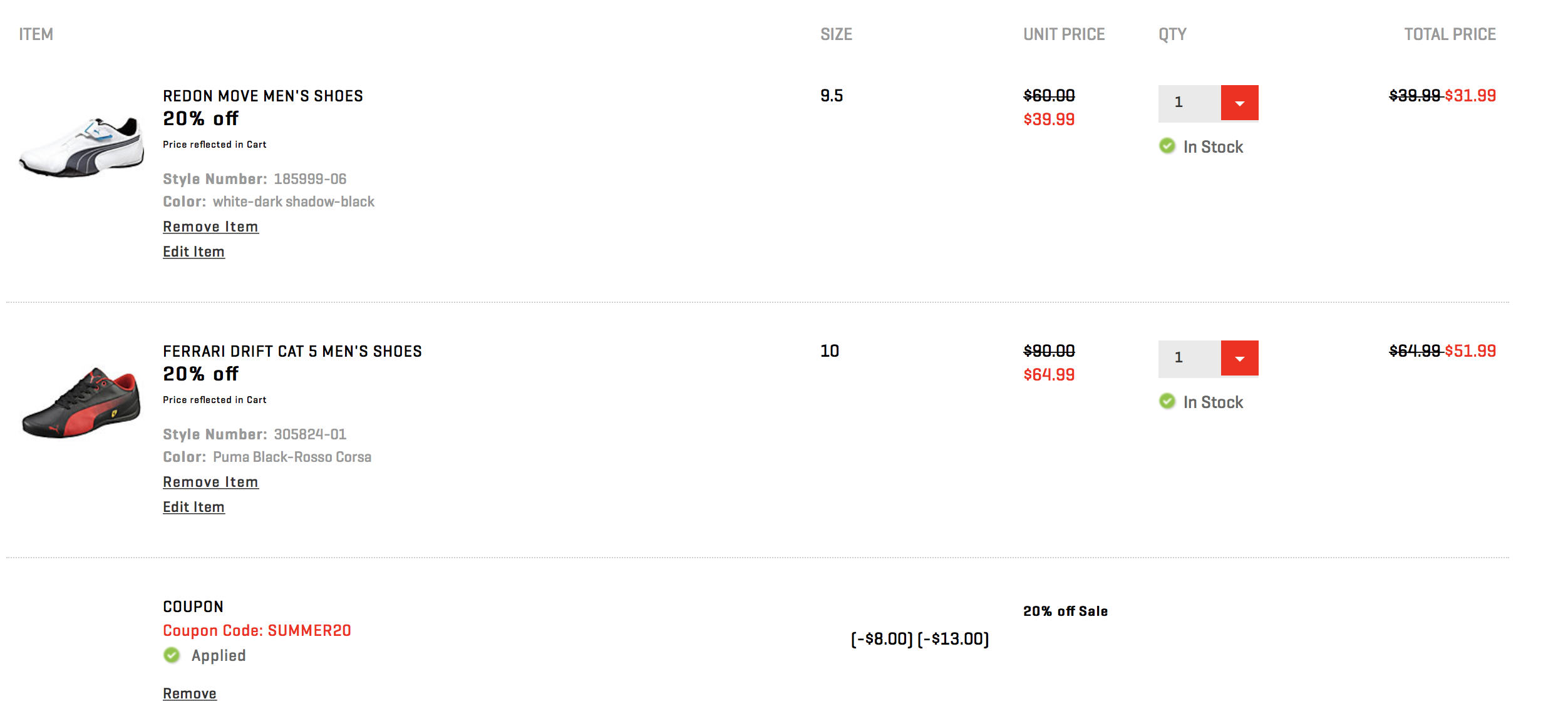The image depicts a shopping cart page from a website dedicated to selling shoes. In the top left corner, the interface displays column headers: "Item," "Size," "Unit Price," "Quantity," and "Total Price." 

Within the cart, there are two distinct pairs of shoes. The first item is the "Red On Move Men's Shoes," currently offered at a 20% discount. It features a style number, color tag, and options to either remove or edit the item. This pair is available in size 9.5, originally priced at $39.99, but with a discount, the total price is reduced to $31.99.

The second item in the cart is the "Ferrari Drift Cat 5 Men's Shoes," characterized by its black color with a distinctive red stripe. This pair is also discounted by 20%, available in size 10. Initially priced at $64.99, the discount lowers the total to $51.99. 

Located at the bottom of the screen is a section indicating the application of the coupon code "SUMMER20," which has provided the 20% discount applied to both items in the cart.